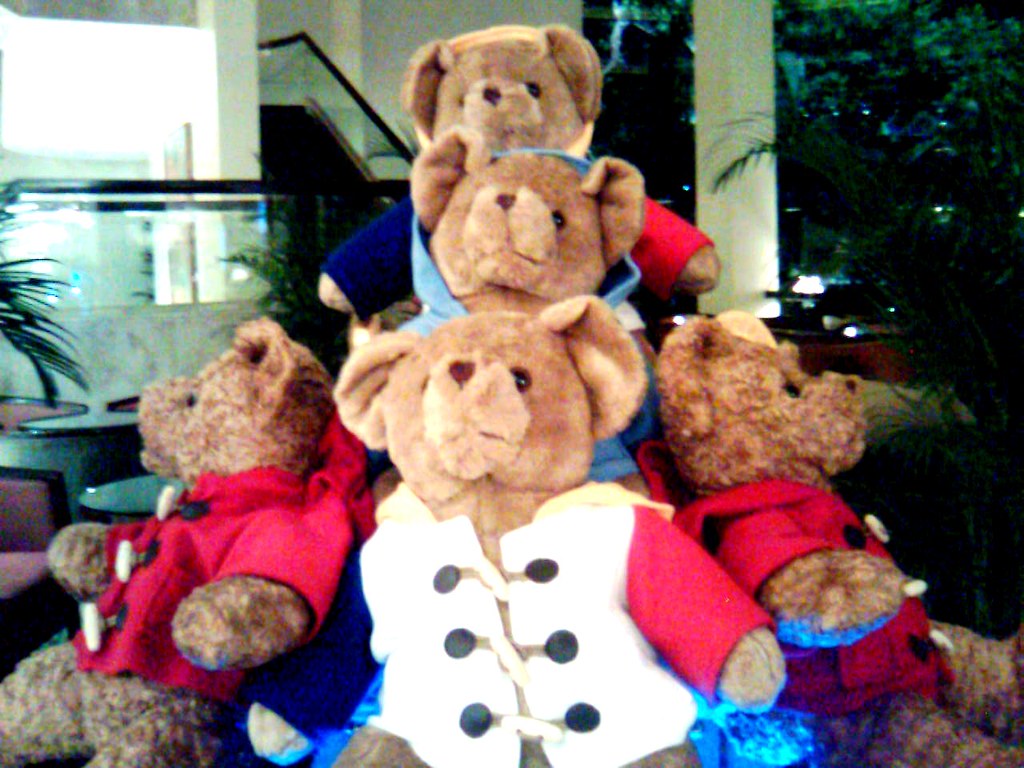In this detailed image, five brown teddy bears are arranged in a room that appears to be part of a house or possibly a restaurant, with a staircase and a table with pinkish chairs outlined in black in the background. The scene features intricate details of each bear’s attire and position. The central teddy bear, dressed in a white jacket with navy blue on the right sleeve and red on the left sleeve, has black buttons down the front. Flanking this bear, one on each side, are two more teddy bears in red shirts adorned with black and white buttons; we see them from a side view. Behind the central bear are two others, partly obscured, but one sports a blue hood and the other has arms with mismatched red and blue sleeves. All five bears have button-like noses and appear to be neatly stacked, creating a layered arrangement where each bear's head is visible above the one in front. Off to the right side in the room, there's a floor plant adding a touch of greenery to the scene.